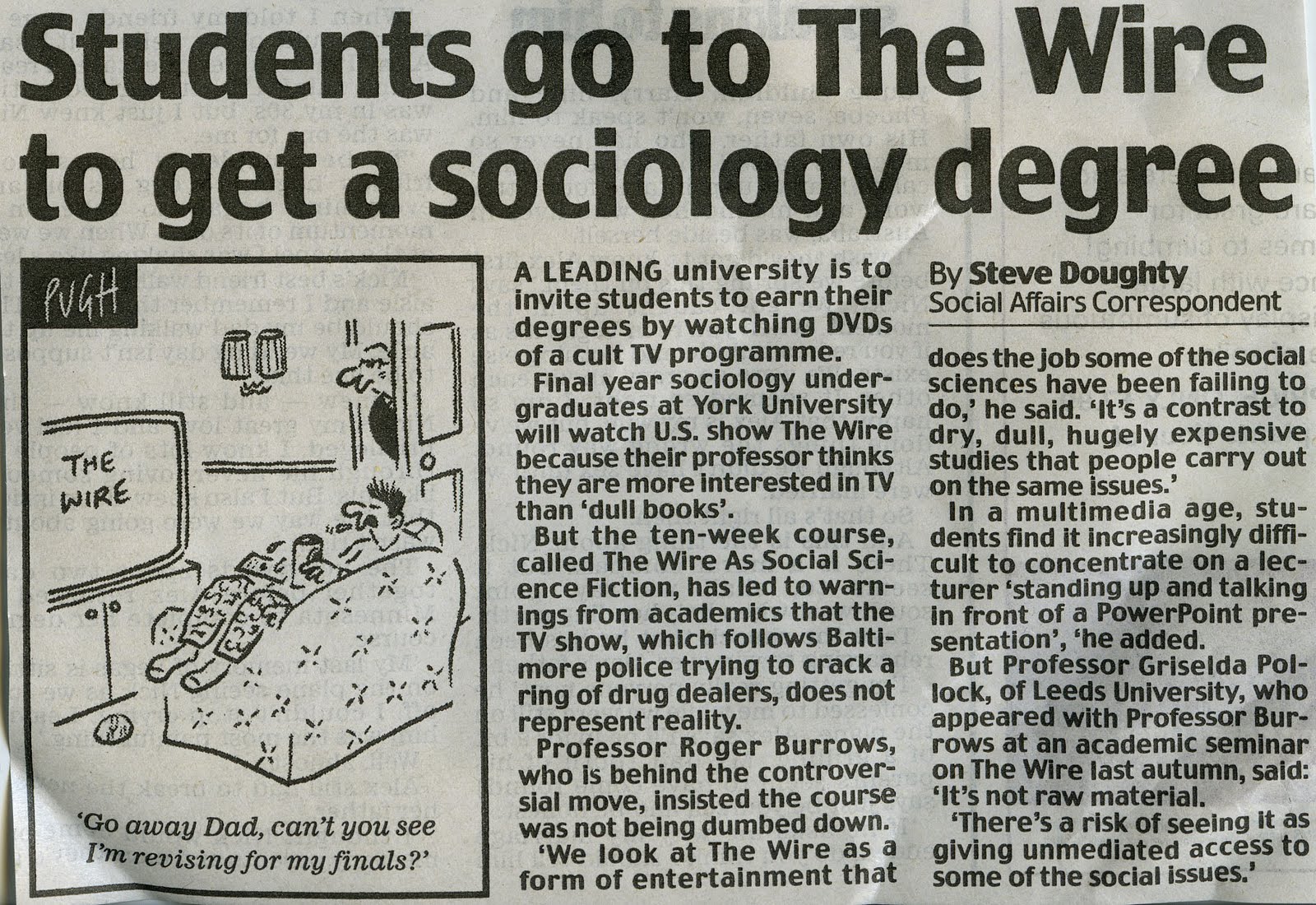This image is a clipping from an actual physical newspaper, recognizable by its bent corner and visible creases. Additionally, the faint outline of text from the reverse side of the clipping can be seen through the paper. The clipping features an article titled "Students Go to the Wire to Get a Sociology Degree," written by Steve Daughtry, the social affairs correspondent.

Accompanying the article is a cartoon illustration depicting a boy lounging on a sofa, engrossed in watching "The Wire" on television. An adult, likely his father, stands in the doorway, observing the scene as the boy munches on popcorn. The cartoon's caption reads, "Go away, Dad. Can't you see I'm revising for my finals?" This visual humorously suggests that the television show "The Wire" possesses significant educational value, particularly for students studying sociology. The article discusses initiatives by leading universities to incorporate watching DVDs of the cult TV program as part of earning a sociology degree.